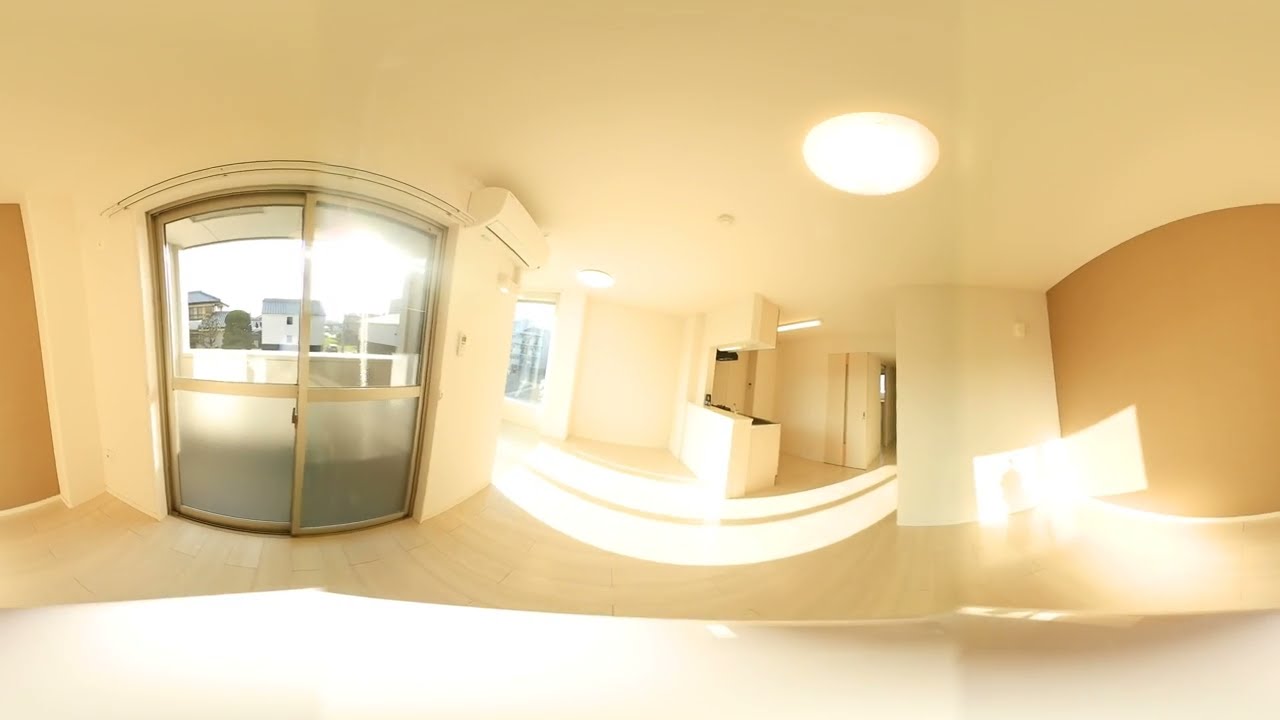The image depicts a bright and vacant apartment with a warped, panoramic view. The room shows plenty of natural light filtering through sliding glass doors on the left, which open to a white balcony overlooking a residential neighborhood. The day appears overcast from the glimpse outside. The walls inside are mostly white, except for a distinctive curved wall on the right, which has a gold hue. The flooring is composed of light tan or wooden planks that add to the airy ambiance. 

Ceiling lights include a mix of circular fixtures and a fluorescent tube light, likely situated in the kitchen area. The kitchen features an island or breakfast bar with room for bar stools, along with a hood fan visible on the left side. There's a nook that could serve as a dining area beside the sliding doors. This kitchen area, although missing appliances like a stove and refrigerator, includes tall cabinets and showcases an open front design suitable for bar seating. The overall bright and empty space, with its varied wall colors and light wood flooring, contributes to a modern and expansive feel.